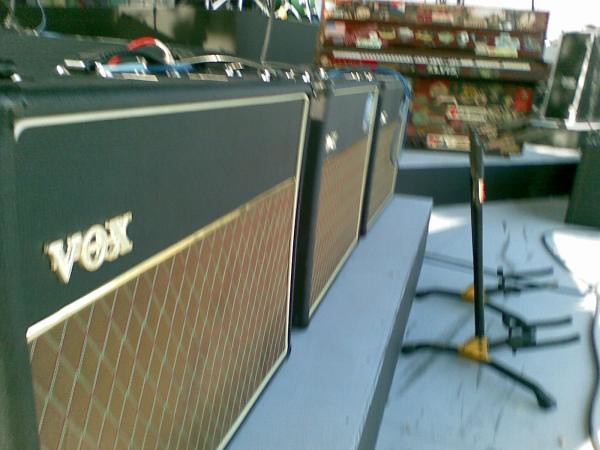In the foreground, we see three vintage-looking box amplifiers with a suitcase style, marked with the brand "VOX" in white letters on a dark green surface and adorned with a diamond-shaped brown pattern indicating the speaker area. These amplifiers, which are commonly used for electric guitars, are elevated on a light blue, blue-green stand. Slightly out of focus, there's a stand configured to hold a guitar. Surrounding these items, possibly resembling a music store, the scene is slightly blurred but includes additional stands and a variety of musical equipment. To the left, there's a handle on the amplifier-like structure, and cables in red, black, and blue are visible. In the background, barely discernible shelves and a piano with memorabilia are displayed, adding to the cluttered yet authentic ambiance of the store-like setting.